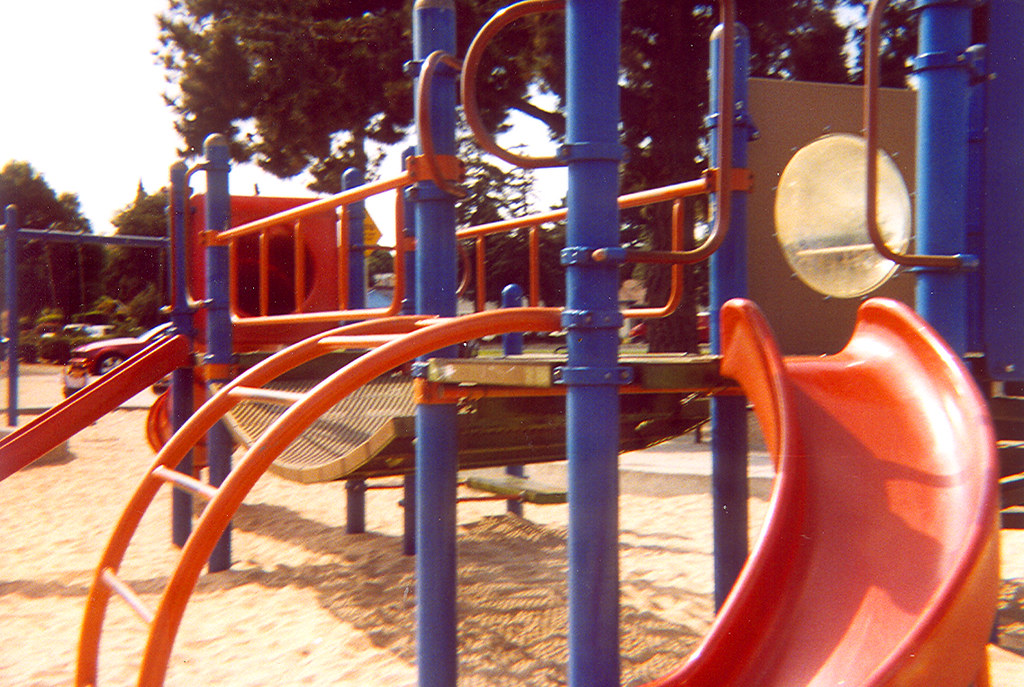The photo captures a vibrant, outdoor children's playground, set on a sandy lot which gives it an older appearance with its somewhat faded colors. Dominated by various play structures, the scene is anchored by a prominent orange slide on the right that curves gracefully to the ground. Adjacent to the slide, an orange ladder mirrors the curvature, offering a path for climbing. 

A small, rounded window in gray or brown, perfect for peeking through, sits to the right of the slide. The playground also features a yellow swinging bridge that connects two elevated platforms, inviting children to traverse between different play areas. On the left side, another climbing structure appears, with blue support beams adding a touch of cohesion to the entire setup.

Behind the primary play structures, there is an additional play area that includes a swing set and another slide that is partially obscured due to the distance and angle of the shot. Surrounding the playground, a large fence adds an element of safety, while a red truck and a large tree can be seen in the background, providing context and depth to the scene. An overcast blue sky forms the backdrop, giving the playground a timeless and inviting feel, with the hint of a red car and a glimpse of a child nearby enhancing the sense of active play.